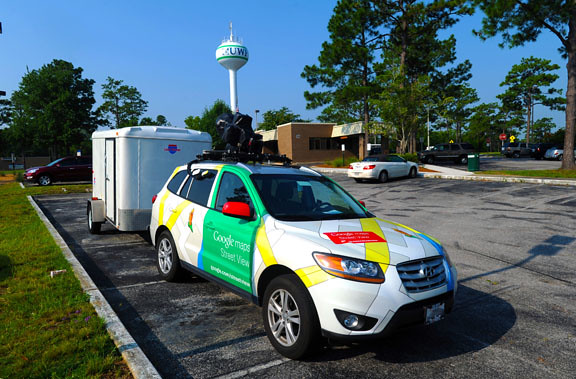The image captures a vibrant outdoor scene in a public parking lot under a clear, bright blue sky. Central to the image is the distinct Google Maps vehicle, a white hatchback adorned with a green passenger door, a red side mirror, and a map-like design featuring yellow lines representing roads. This car, identified as a Hyundai, prominently displays the Google Maps Street View logo on the side. Atop the vehicle is the familiar camera equipment used for capturing street views. The Google Maps vehicle is also towing a white trailer, presumably for additional equipment. To the left of the vehicle, a cement curb transitions into a grassy area.

In the background, a variety of elements are visible, including a white water tower with blue stripes and letters "K-U-W," green trees, and a brown brick building that appears to have a drive-thru, possibly a bank. Additional details include a red stop sign, a yellow diamond-shaped traffic sign, and another white car with a black top parked further back and to the right of the Google Maps vehicle. The parking lot itself is made of gray cement and features multiple parking spaces, with the overall scene bathed in bright natural light.